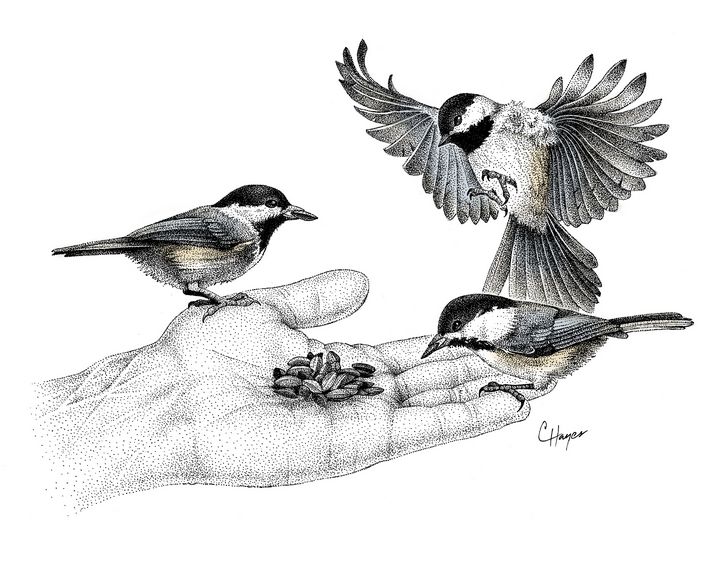This detailed pen and ink drawing, signed by the artist in cursive as "Sea Hamper" in the bottom right corner, captures a calm and serene moment of three birds feeding from a man's outstretched hand. The hand, prominently featured and cropped at the wrist, displays visible veins and creases, extending from the left side of the paper. In the center of the man’s light-colored palm lies a collection of what appear to be sunflower seeds. 

The three birds, likely of the same species and resembling small sparrows, exhibit subtle coloration with a predominantly black-and-white palette and faint hints of light brown or yellow. One bird is perched serenely on the man's thumb, another is balanced on his pinky finger, while the third bird is captured in mid-flight, its wings outstretched as it prepares to land, possibly on either the index or middle finger. Notably, two of the birds already have seeds in their beaks, indicating their mid-action in feeding, while the third is yet to start. The overall composition is detailed and tranquil, with the birds appearing calm and relaxed against the stark, white background.